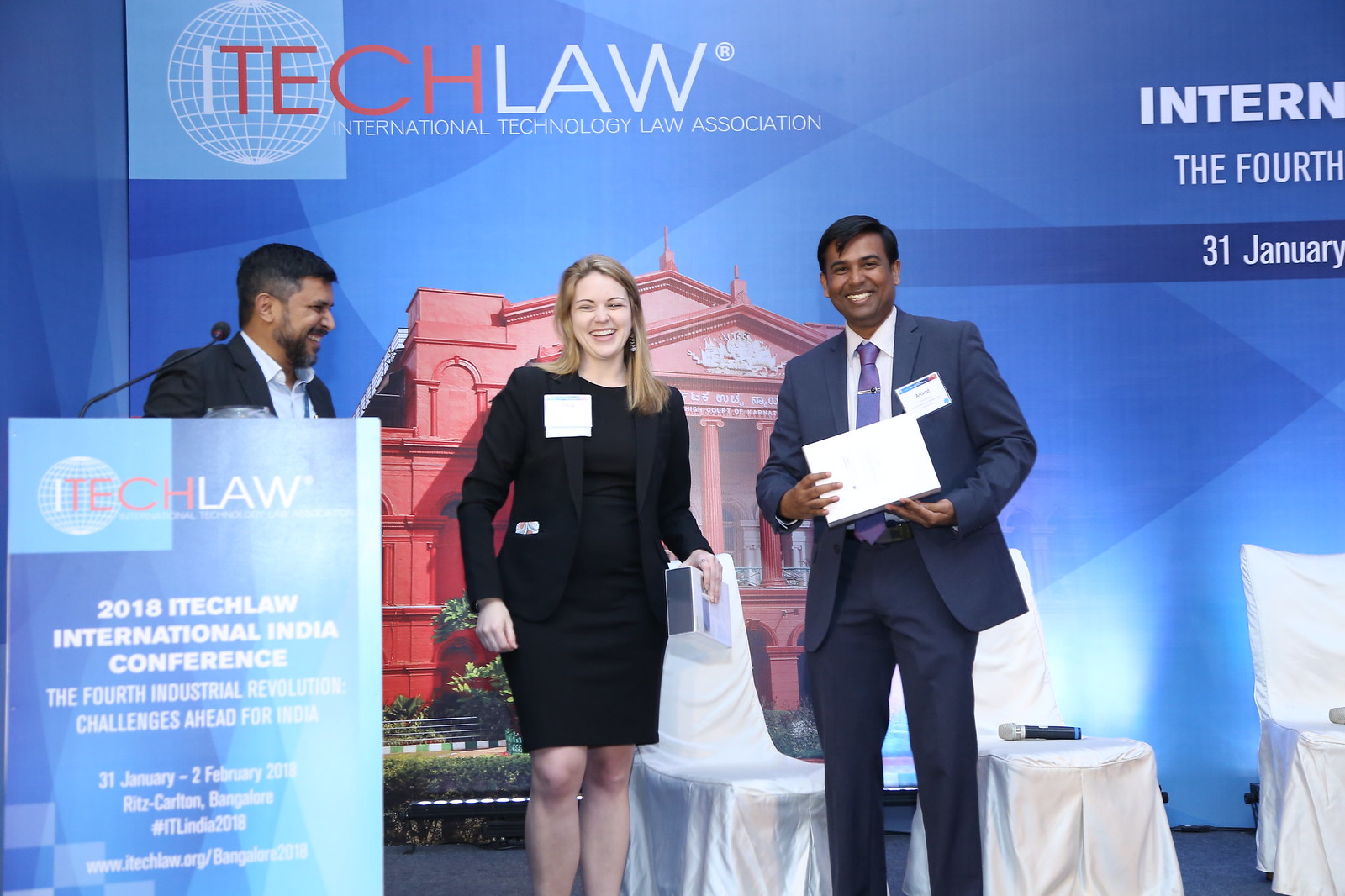The photograph captures a moment at the 2018 I-Tech Law International India Conference, focusing on challenges posed by the Fourth Industrial Revolution. Three individuals stand on a stage against a blue backdrop featuring the I-Tech Law logo, a stylized globe, and partially visible text "International Technology Law Association." The backdrop also includes an image of a classical building with columns. Positioned centrally is a young Caucasian woman with blondish hair, dressed in a conservative black dress and wearing a name tag, smiling at the camera. Flanking her are two men of darker complexion; to her left is a dark-skinned man with a beard, and to her right, a young South Asian man in a suit, also wearing a name tag, holding an award sign or plaque that partly cuts off another figure in the lower left corner. A podium with the Tech Law insignia stands before the woman, and three chairs covered with sheets and a microphone are visible behind them, suggesting they are poised to address the conference. Red and white lettering on the backdrop highlights key details: "The Fourth Industrial Revolution," "International," "31st January," emphasizing the importance and timeliness of the event.